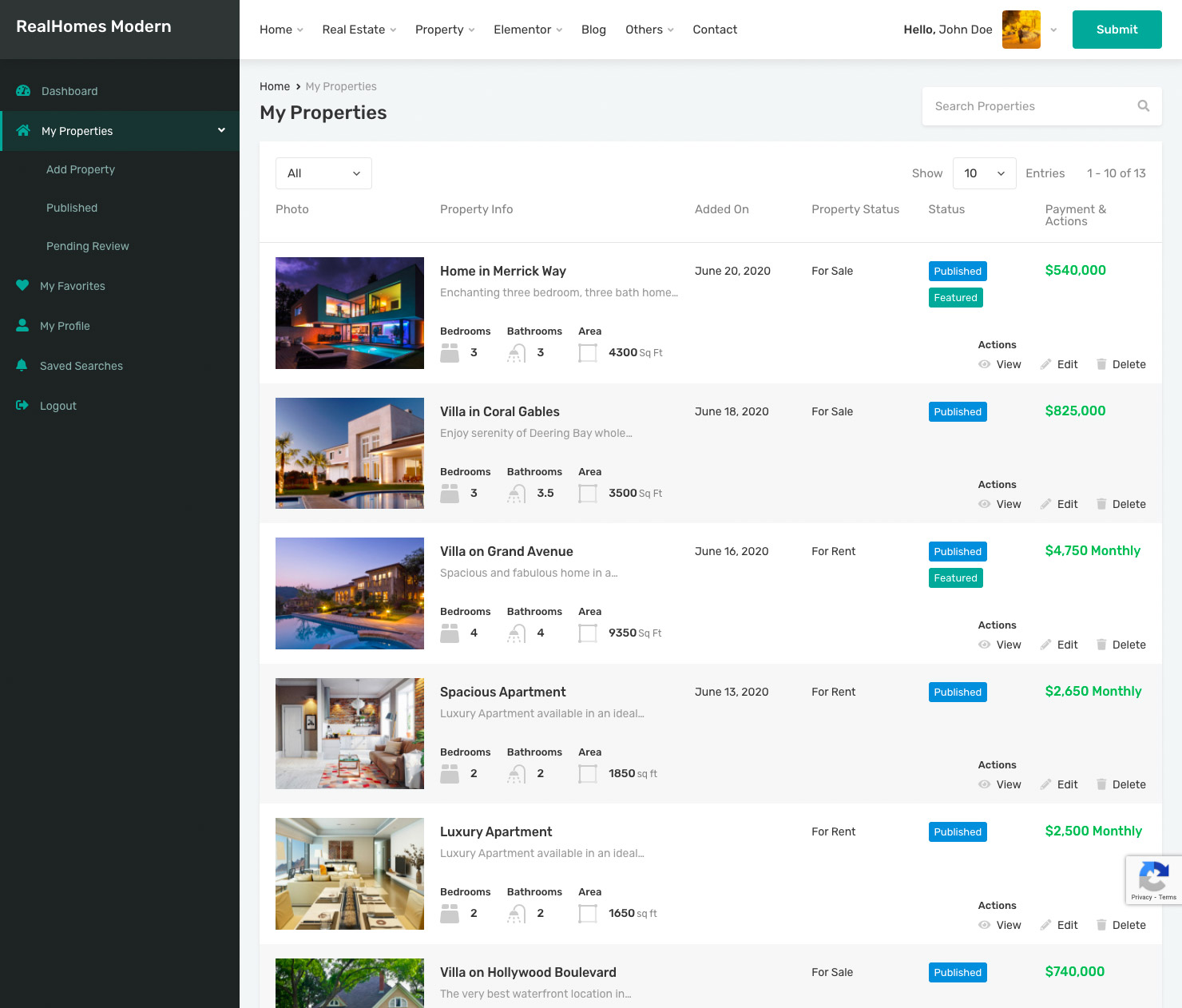The image depicts a comprehensive webpage layout for the "Real Homes Modern" platform. Located in the top left corner, a light gray box displays the "Real Homes Modern" title, with a separating line running vertically down the page. Below the title, the left-hand side features a navigation panel set against a black background. This panel includes:

1. Dashboard (with an icon beside it)
2. My Properties (highlighted with a house icon, and a drop-down arrow revealing options like Add Property, Publish, and Pending Review)
3. My Favorites (denoted by a heart icon)
4. My Profile (accompanied by a profile icon)
5. Save Searches (represented by a bell icon)
6. Logout (indicated by a logout icon)

In the central part of the page, the heading "My Properties" stands out. On the right, there's a "Search Properties" box featuring a search icon.

Below this, the page lists six property selections. Unfortunately, the sixth property's details are partially cut off. The property list section is organized with headers such as:

- Property Title (e.g., "Home in Merkway" is the top listing)
- Dates
- Property Status (e.g., for sale, for rent)
- Payments
- Actions

Near the bottom right corner, there is a "ReCapture" button.

Overall, the webpage appears to be a user dashboard for managing property listings with a functional layout for ease of navigation and property management.